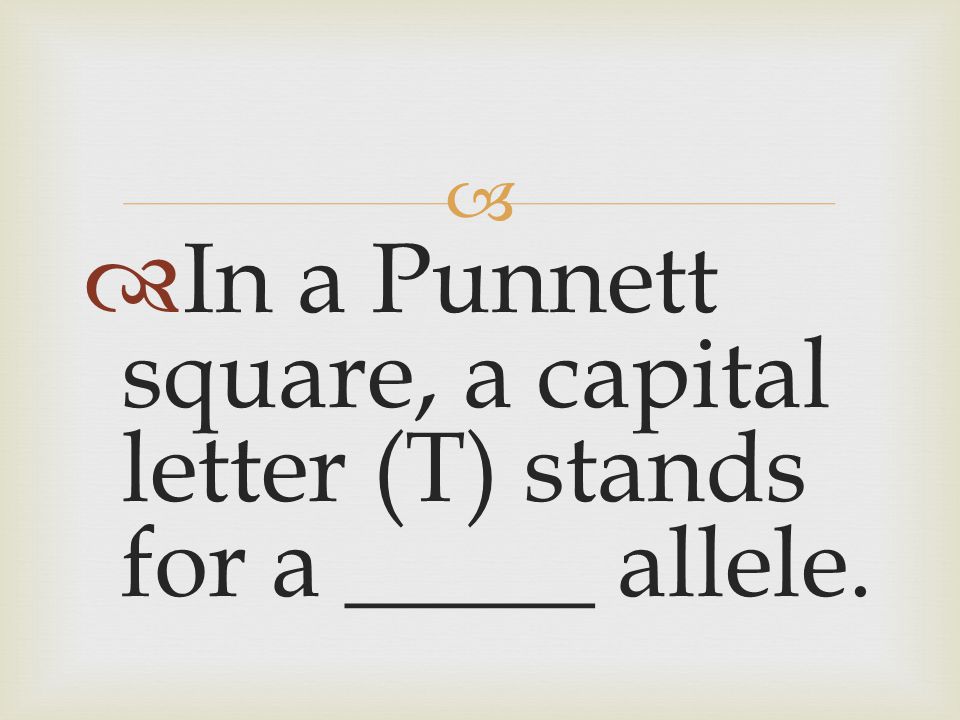The image features a white background framed by a thin light yellow or golden border. Centered on the image, there is a decorative design that includes a small orange line and a partially visible red flower or flowery design on the left side. Prominently displayed in black text is the phrase: "In a Punnett square, a capital letter (T) stands for a blank allele." The letter "T" is capitalized and enclosed in parentheses, followed by a blank underscore for someone to fill in with the correct answer. The text is neatly formatted with each phrase centered on separate lines, and the overall composition maintains a clean and organized appearance.